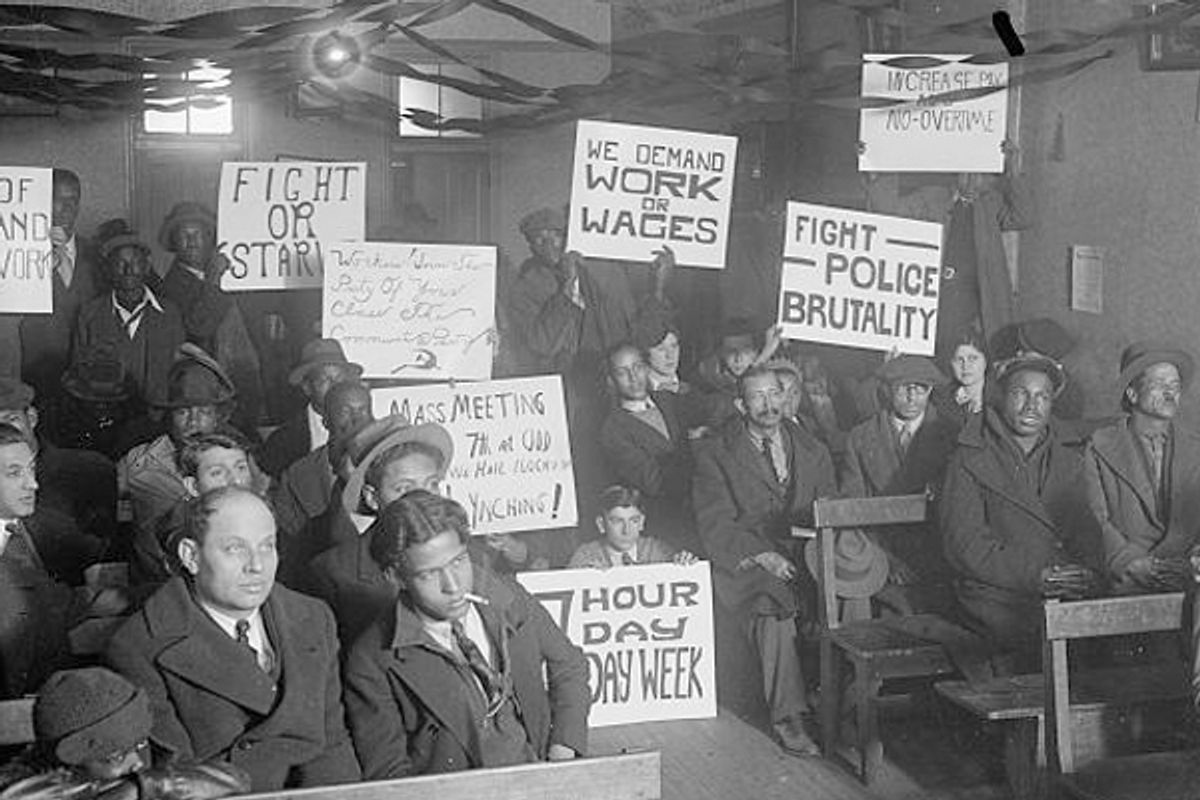In this black-and-white photograph, an organized assembly of primarily African-American men, with a few women, is seated on benches in what appears to be a public meeting room. The attendees are dressed in long, dark coats, suggesting it is winter. They are all facing forward, seemingly attentive to something outside the frame. Approximately 20-25 individuals are present, most of whom are of working age, and they hold various protest signs. The signs bear slogans such as "Fight Police Brutality," "We Demand Work or Wages," "7-Hour Day Week," and "Fight or Starve." A notable figure at the front has a cigarette dangling from his mouth. The atmosphere in the room is charged with unified determination, indicating a collective effort to voice socio-economic grievances, likely in a government or board meeting setting.